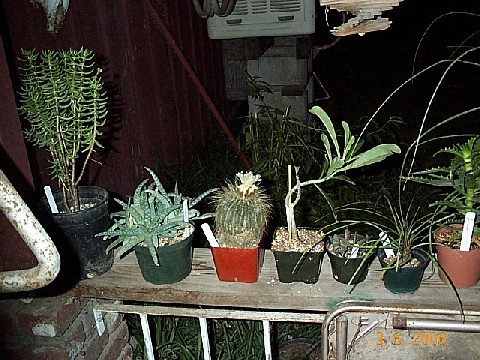The photograph depicts a nighttime scene in what appears to be someone's backyard. A row of eight potted plants, varying in size and type, sits on a wooden plank that rests atop a metal railing or gate. On the left side of the picture, a brownish-red wooden fence is visible along with a metal contraption near the fence. The plants, illuminated by artificial lighting from the camera flash, include a mix of succulents, cacti, and other desert plants. The largest plant on the far left is a tall, green-leafed bush in a black pot. Following that is a smaller, star-shaped green-leaf plant in a green pot and a classic-looking cactus in a red pot. Next is a curious plant with a long branch and a flower-like end, situated in a black pot. This is followed by a circular black pot containing what seems to be a dead plant. To its right is another bush-like plant with green leaves in a green pot, and finally, a tall, green-stemmed plant in a red pot occupies the far right. The background is almost entirely dark, emphasizing the plant arrangement. A date mark reading "3-6-2006" appears in orange in the bottom right-hand corner, indicating when the photo was taken.